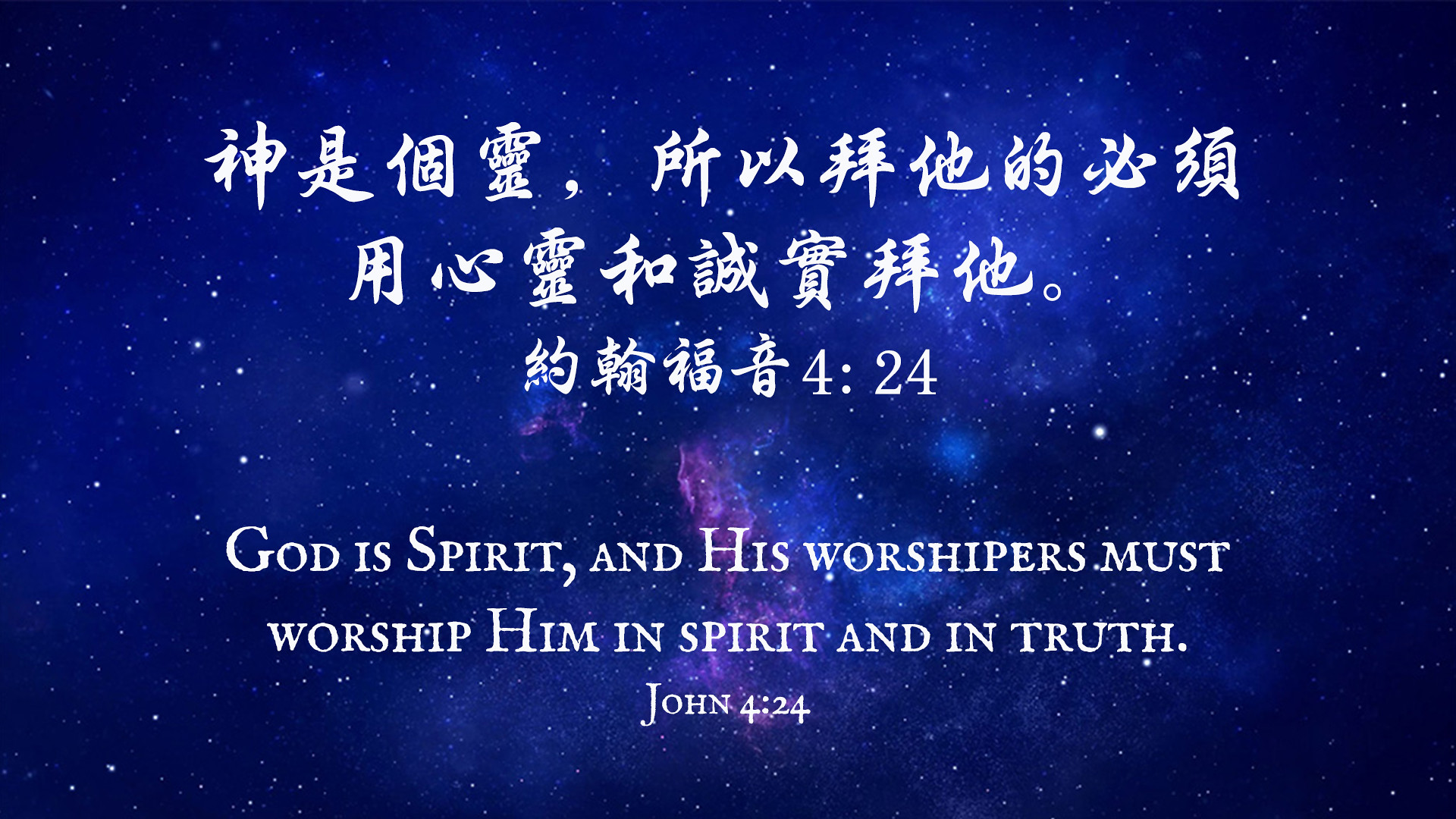The image features a vibrant depiction of the night sky, intricately detailed with a galaxy that spans the background, blending shades of dark blue, purple, light blue, pink, gray, and white. Scattered across this celestial canvas are numerous white stars, with one particularly bright star positioned slightly to the right of the center. Dominating the top portion of the image are three lines of Chinese characters, elegantly rendered in white. Below the Chinese text, centered in English, is the scripture quote: "God is Spirit, and His worshipers must worship Him in spirit and in truth. John 4:24," with meticulous emphasis on capitalization and punctuation. Together, the celestial background and the bilingual scripture create an inspiring, spiritual composition designed to evoke a sense of faith and awe.